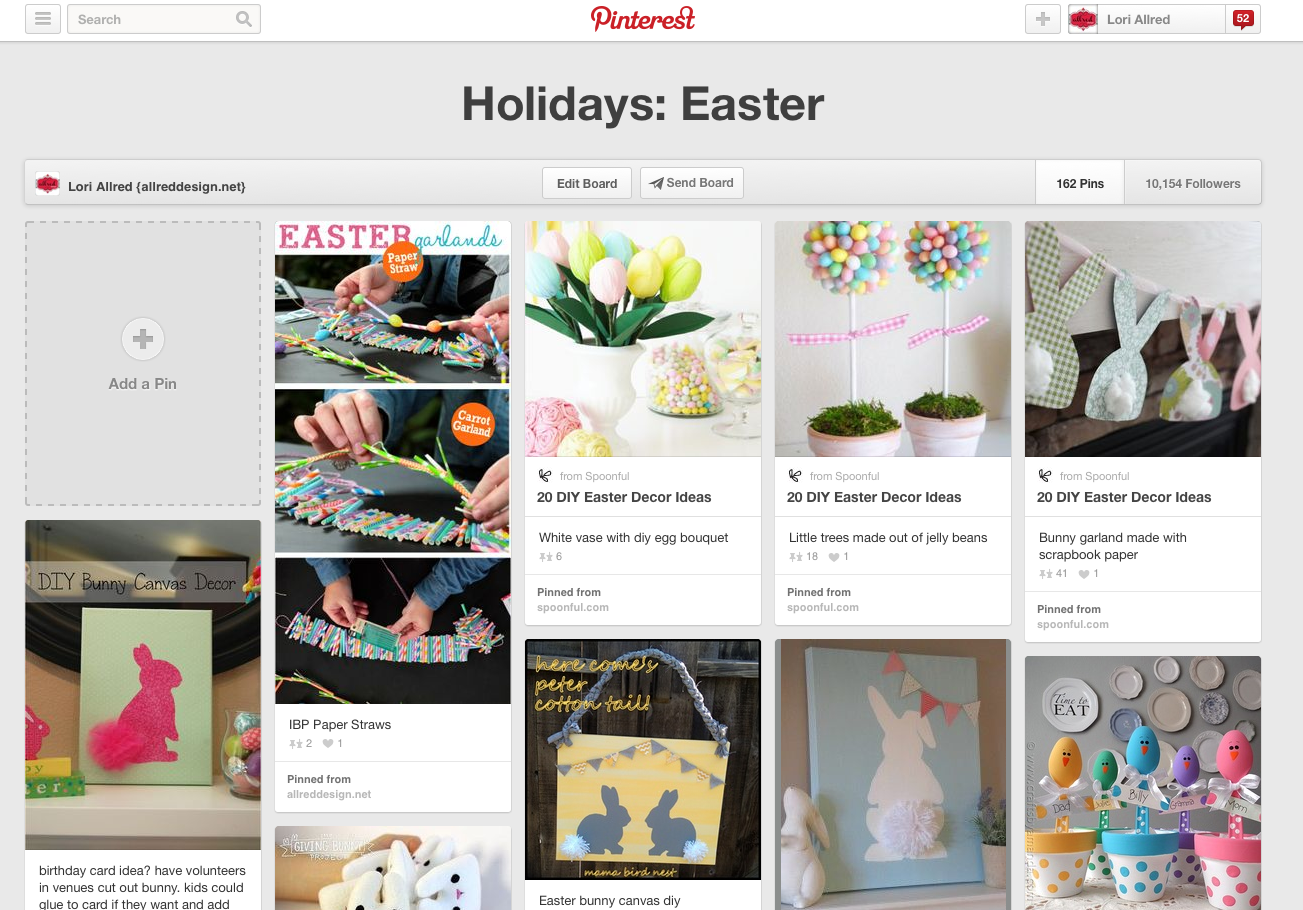Here's a refined and highly detailed caption for the image:

---

The image showcases a Pinterest page titled "Holidays: Easter," featuring bold black lettering at the top. At the upper section, the page identifies the curator, Laurie Allred from allreddesign.net, with a small thumbnail representing her business. Positioned along a central banner, there are interactive buttons labeled "Edit Board" and "Send Board," with the latter marked with a send icon. To the right of this banner, the board's statistics are displayed: "162 pins" and "10,154 followers."

In the first row of images, the initial space features a blank gray area with a plus sign and the text "Add a Pin." Following this, a vibrant photo depicts the creation of "Easter Garlands" with pink and blue text. It includes two snapshots: one showing paper straws being fashioned into a carrot garland, and another displaying the completed garlands, all captioned "IBP paper straws pinned from allreddesign.net." The subsequent pin highlights "20 DIY Easter Décor Ideas," featuring a white vase filled with a DIY egg bouquet, accompanied by jars of candy and a variety of flowers. Next, another pin presents decorated whitewashed terracotta pots filled with moss and topped with pastel-colored Easter egg clusters, with pink and white gingham ribbons tied around the stems. Adjacent is an image showing a ribbon adorned with four patterned Easter bunny silhouettes with cotton tails, also labeled "20 DIY Easter Decor Ideas."

The second row opens with a pin captioned "DIY Bunny Canvas Decor," showing a light green frame with a pink bunny silhouette, featuring a loofah used as the bunny's tail. Additional text suggests a birthday card idea involving volunteers and venues for cutting out bunnies that children could glue onto cards. An adjacent pin features a partially visible image of stuffed animals. Following this, another pin with a dark background presents a handmade sign of two gray rabbits with fluffy tails, accompanied by the caption "Easter Bunny Canvas DIY" and the text "Here Comes Peter Cottontail" in yellow. The next image displays a blue canvas with a white Easter bunny silhouette from the back, complete with a pom-pom tail, and paired with an Easter bunny statue. The last image in the second row shows three pastel-colored pots with polka dots, each appearing to grow eggs painted like chicks in green, yellow, blue, purple, and pink, all set against a backdrop of decorative plates on the wall.

---